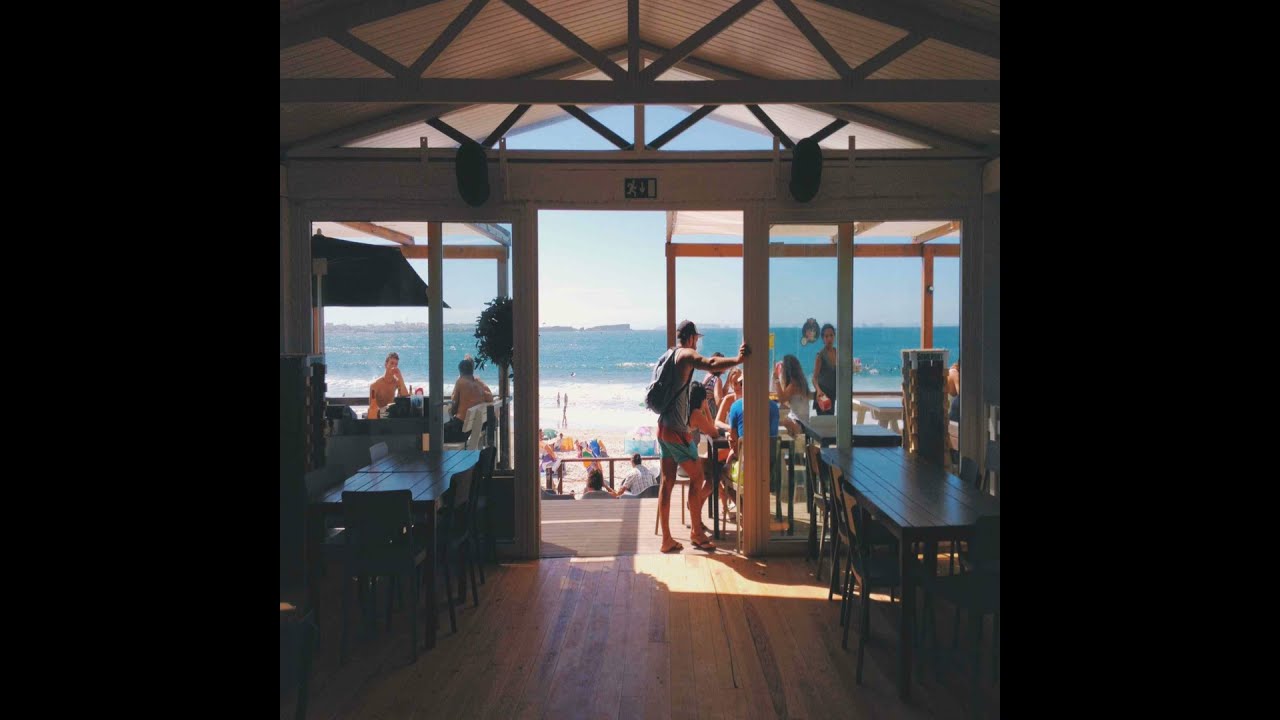The image depicts a vibrant beachside scene viewed from within a cafe or restaurant. The photo, almost hyper-realistic, shows a spacious interior with wooden tables and chairs arranged on dark wooden floors. The ceiling features exposed beams, adding to the rustic charm. The large, open doorway and floor-to-ceiling windows flood the interior with sunlight, revealing a bustling outdoor patio. People are seen enjoying the sunny day, some seated at tables, others standing, and more can be seen farther out on the beach engaging in various activities. In the center of the image, a man leans casually against a pillar, gazing out at the ocean. The scene is dominated by bright hues: the deep blue of the ocean, the white sandy beach, and the distant hills or islands on the horizon. No one is inside the restaurant, which emphasizes the allure of the sunny, inviting outdoors. This lively setting captures a moment of leisure and enjoyment by the shore.